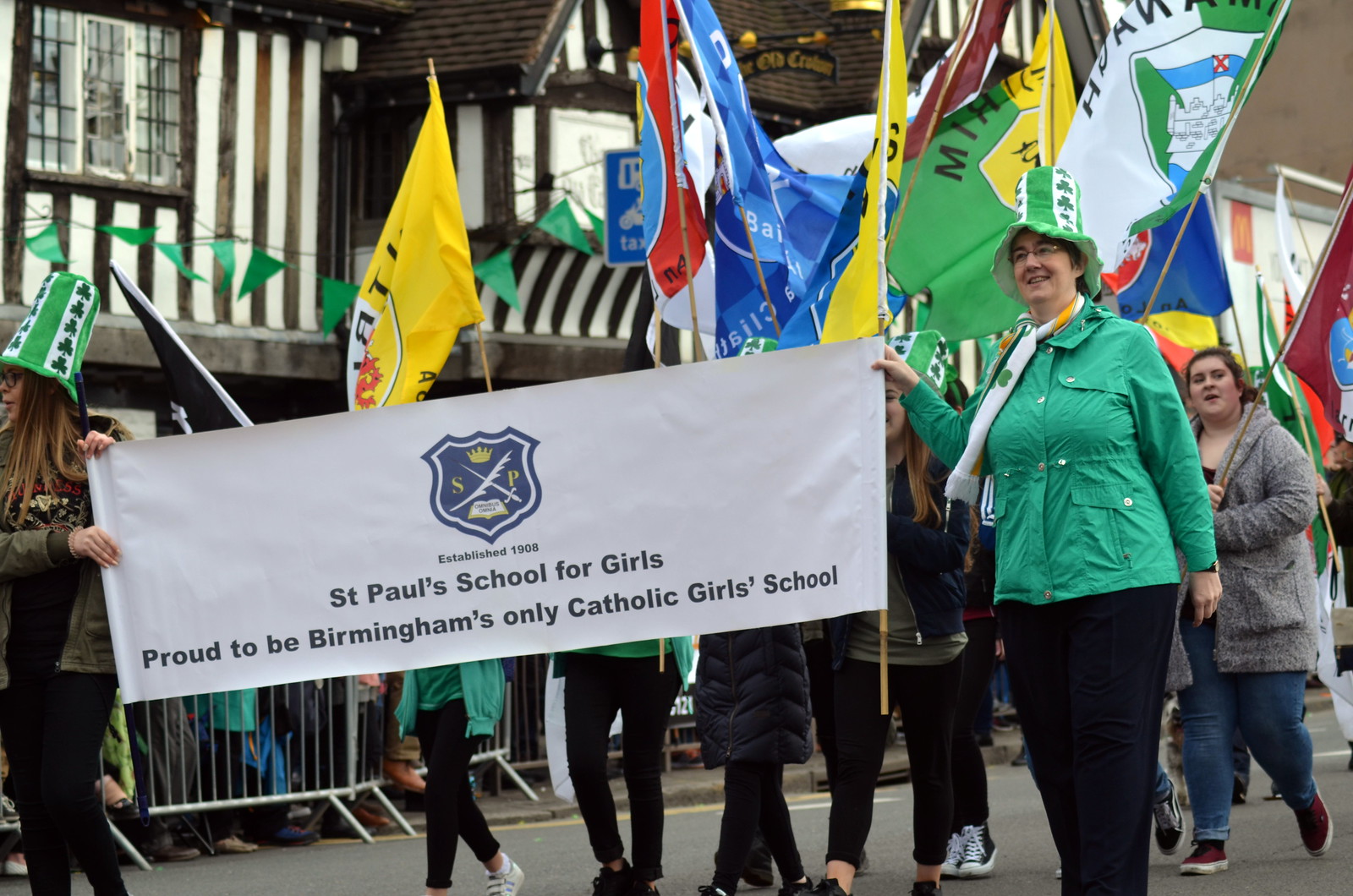In this outdoor daytime photograph, we see a festive parade with a group of women marching proudly down a street. The focus is on a wide, rectangular white banner held by two women at the front. The banner features a shield in its upper half, crossed by a feather and a sword with a crown above, accompanied by the letters "S" and "P" on either side, and a white book below. The text on the banner reads "Established 1968 St. Paul's School for Girls. Proud to be Birmingham's only Catholic girls' school." The woman on the right wears a green shirt and a themed stovepipe hat adorned with vertical stripes and clovers, while the woman on the left is dressed in all black with a grayish jacket and a similar hat. Behind them, a multitude of women, mostly obscured by the banner, carry an array of vibrant flags in colors such as blue, white, green, yellow, red, and more, contributing to the colorful and spirited atmosphere of the parade. The scene is set against a backdrop of older-style buildings with brown and white vertical stripes and crowded windows, and a metal barrier can be seen in the lower left corner, indicating the presence of an audience watching the procession.